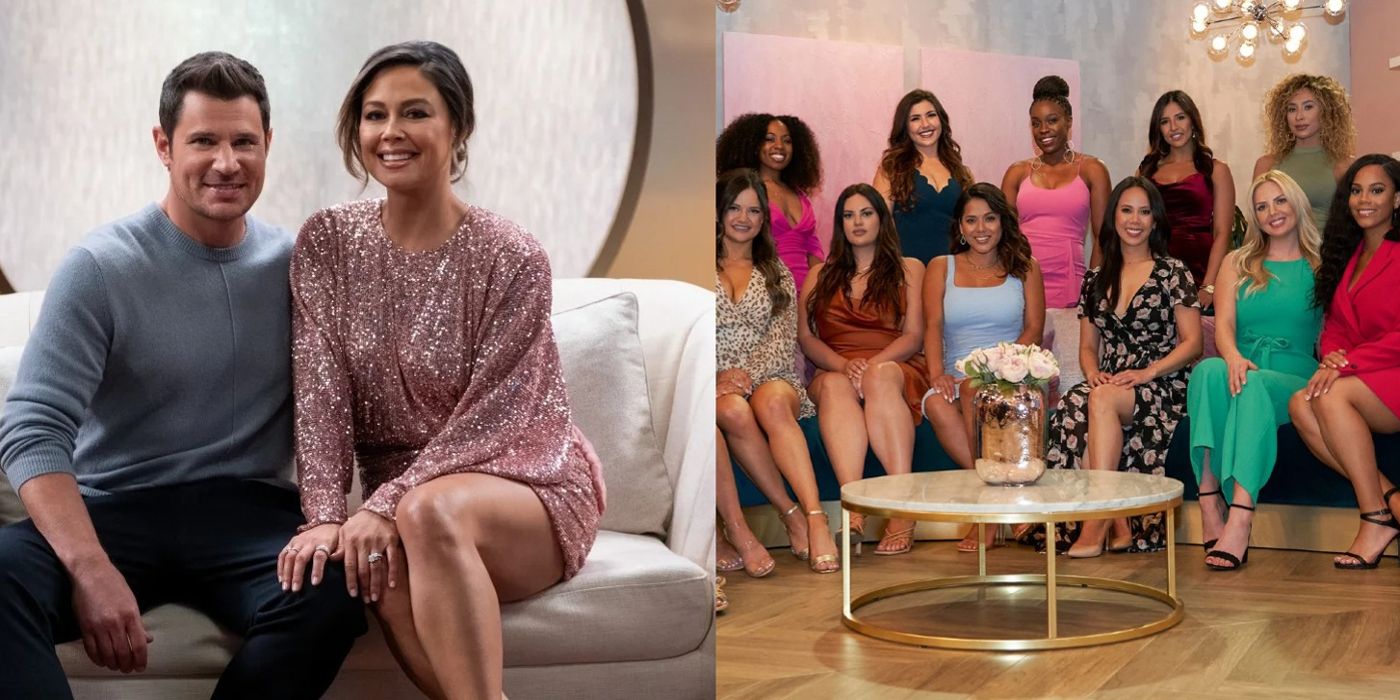This photograph consists of two side-by-side images, possibly from a reality TV show like "The Bachelor." On the left, a man and a woman sit closely on a small white couch, smiling at the camera. The man, who resembles Nick Lachey, wears a stylish light blue long-sleeve shirt paired with dark blue pants. The woman beside him, placing her hand on his knee, is dressed in a sparkly rose-colored mini dress. Behind them, a large circular mirror or art piece adorns the wall, adding a touch of elegance to the setting.

The image on the right showcases 11 women poised in an aesthetically pleasing arrangement: five standing at the back and six seated on a large couch. They are all impeccably dressed in various vibrant dresses and are smiling towards the camera, exuding a sense of excitement and camaraderie. In front, a circular white table with a shiny copper vase displays a bouquet of white roses, complementing the sophisticated atmosphere. The background features a light chandelier and a sheer curtain backdrop, enhancing the room's elegant ambiance. Most of the women have dark hair, though a few blondes and one with curly hair add variety to the scene.